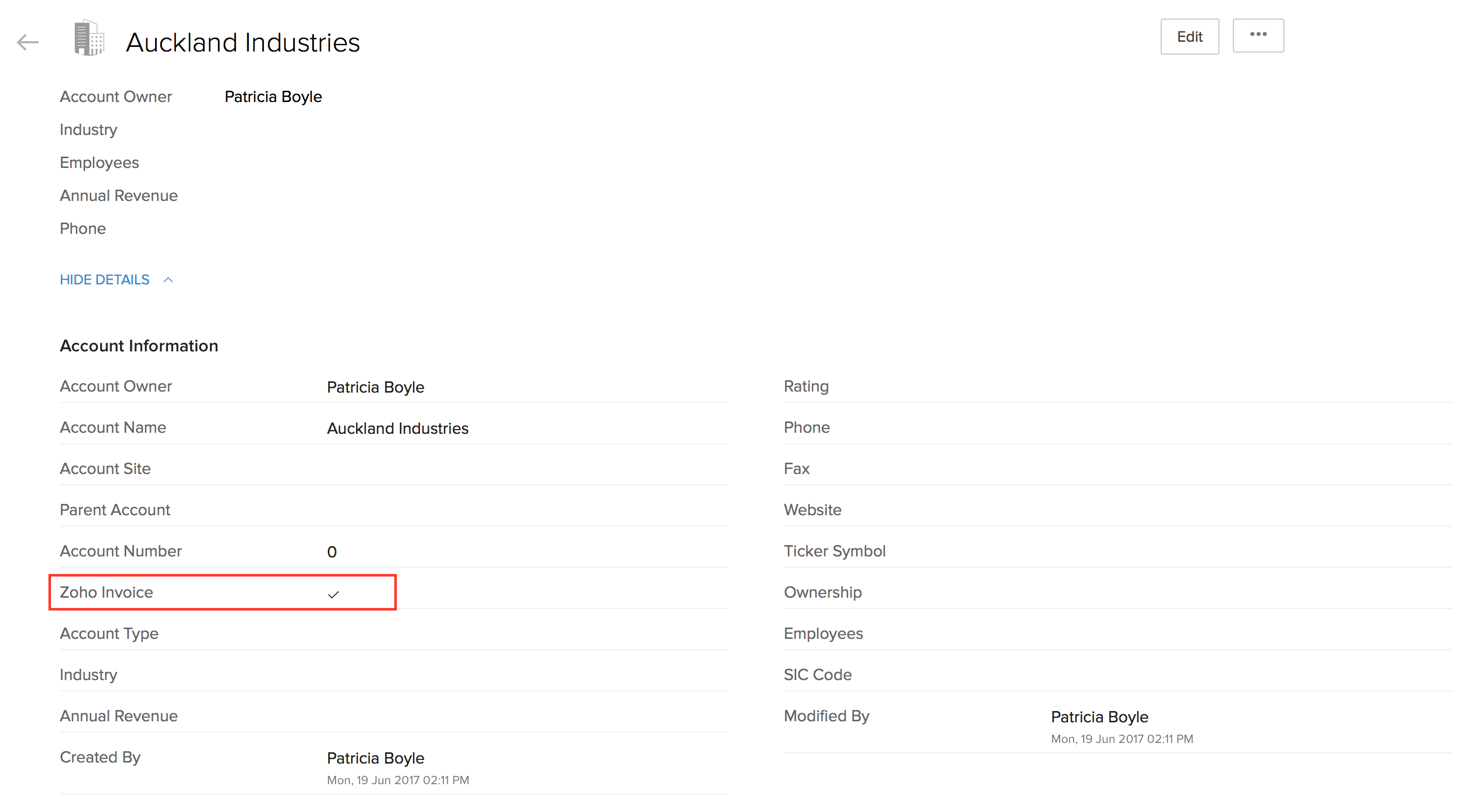**Descriptive Caption for the Image:**

The image displays a detailed view of an account dashboard. On the far left, there is a gray icon representing a building, accompanied by black text. To the right of this icon, the label "Auckland Industries" is prominently displayed. In the top-right corner, there is an edit button with a white background, black text, and a gray outline. Adjacent to this button, an ellipsis icon is situated within a gray-outlined box.

Beneath this section, there is a line of gray text indicating that the account owner is Patricia Boyle, written in black text. Below this personal identifier, there are five lines of information, followed by the label "High Details" in blue text, which is accompanied by an upward arrow. Further down, the text "Account Information" is displayed in black, leading to several rows of detailed information.

Significantly, the fifth row from the bottom features "Zoho Invoice," which is encased in a red outlined rectangle inclusive of a check mark. The name "Patricia Boyle" appears multiple times within the interface: at the top left, middle left, bottom left, and bottom right, signifying her role as the account owner throughout the dashboard.